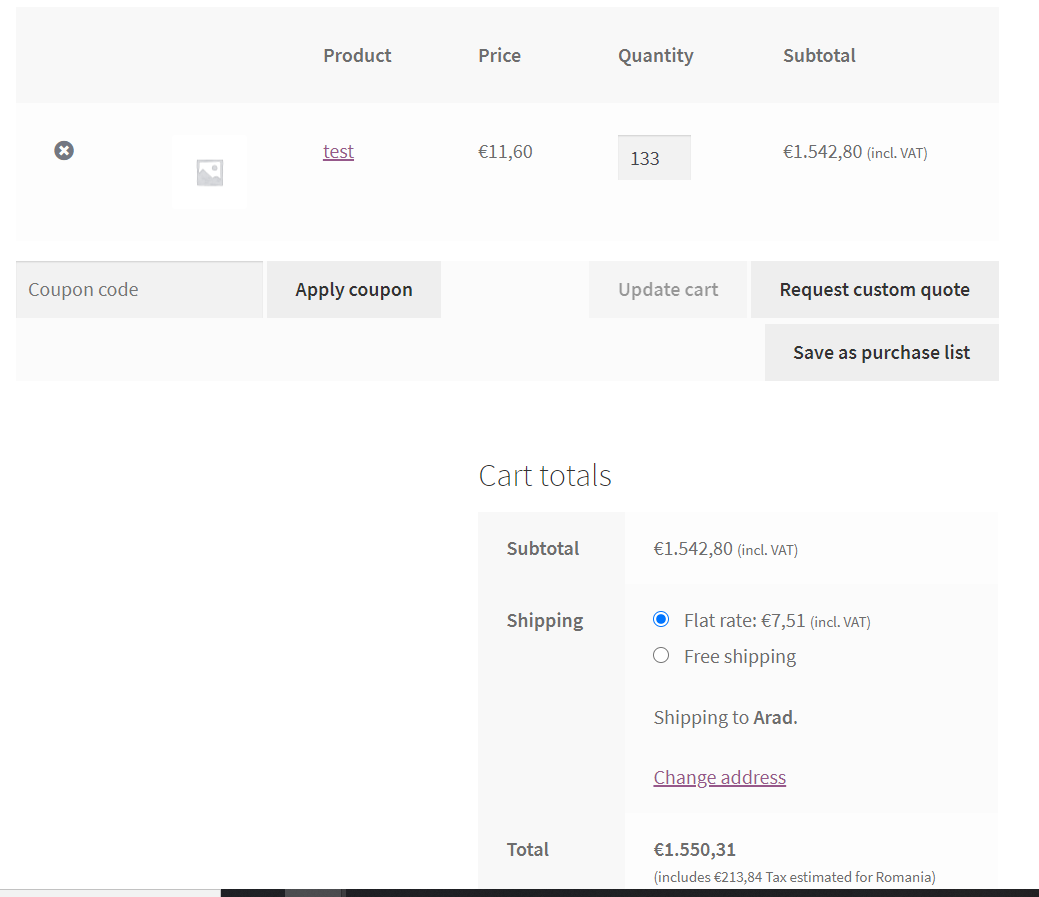The image displays a predominantly white webpage with some gray sections and black text. At the top, headers are labeled "Product," "Price," "Quantity," and "Subtotal." In the first row beneath the headers on the left side, there is an icon representing an image. The adjacent text reads: "Test," priced at 11.60 Euros with a quantity of 133, resulting in a subtotal of 1,542.80 Euros. This amount includes VAT, displayed in Euros.

Further down, there is a field for applying a coupon code, alongside buttons labeled "Update Cart," "Request Custom Quote," and "Save as Purchase List." 

The cart totals section provides a breakdown: the subtotal stands at 1,542.80 Euros, inclusive of VAT. Shipping options are presented, with a flat rate of 7.51 Euros, including VAT, indicated in blue as selected, while the free shipping option remains unselected. 

The total amount to be shipped to Arad (with an option to change the address) is 1,550.31 Euros, which includes an estimated tax of 213.84 Euros for Romania.